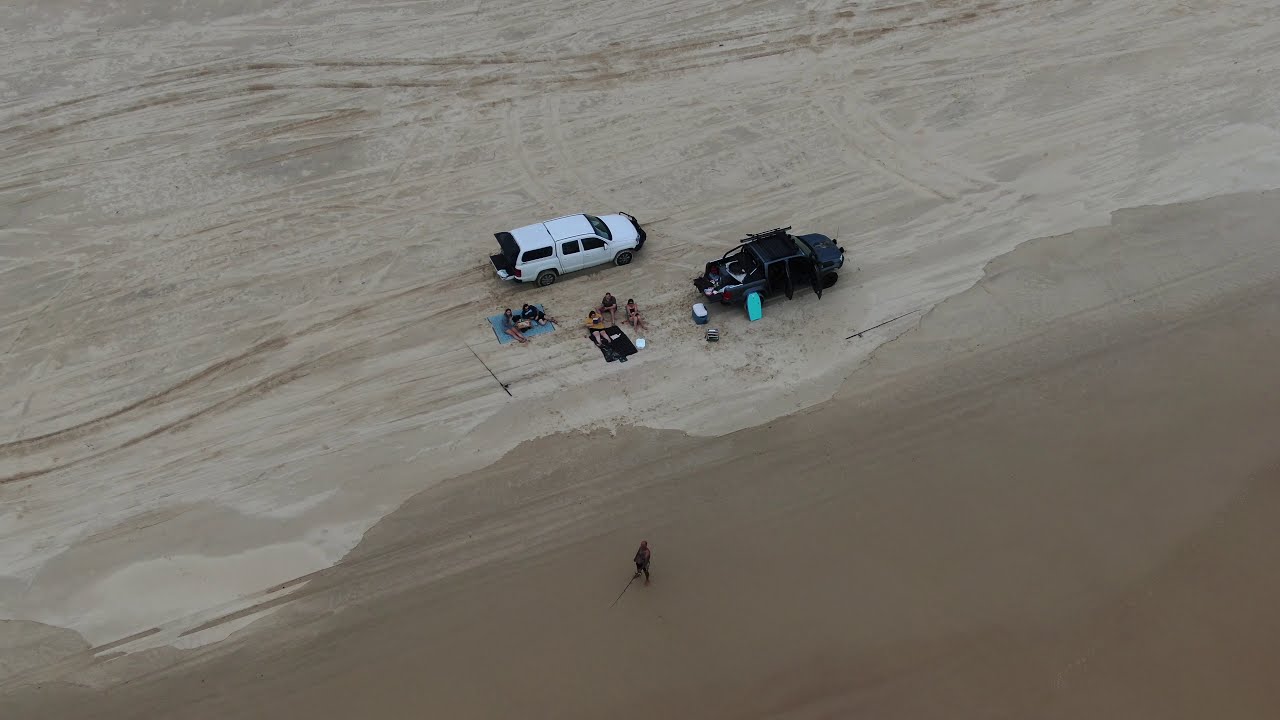This is an overhead photo, likely taken from a drone, capturing a sandy area with no visible water, suggesting it could be a part of a desert or a secluded beach. The sand is two-toned: lighter in the upper part of the image and a darker brownish shade in the lower part. Central to the scene are two families laying on blankets. The families are positioned between a black truck, possibly a Hummer, and a white SUV. Boogie boards or surfboards and fishing poles are leaned against or lying near the black truck, indicating recreational activities. The image also shows tire marks crisscrossing the sand, suggesting recent vehicle activity. A person holding a fishing rod stands a short distance away from the groups, adding a touch of solitude to the scene. The overall color palette includes various shades of brown, white, black, and blue. No text is present in the image, and the absence of the sky focuses the viewer's attention entirely on the sandy expanse and the human activity within it.